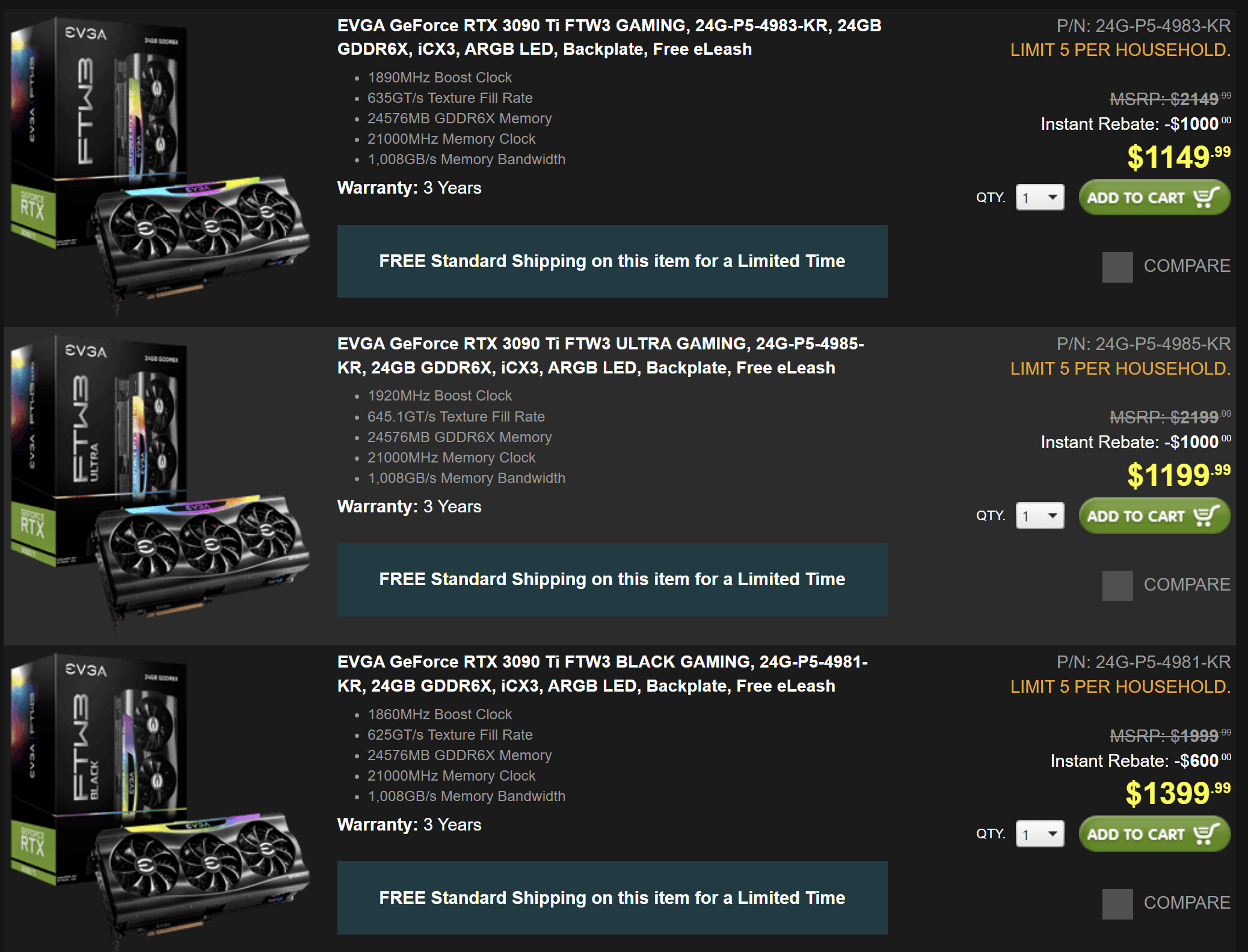The image is a large square divided into three horizontal sections. The top and bottom sections have a black background, while the middle section has a dark gray background. Each section displays the same image on the left-hand side, featuring a product labeled "EVGA FTW3." The image shows a box standing upright with part of the box or another section leaning against it, suggesting it is a type of gaming system.

Beneath the product image in each section, there is descriptive information in white text, detailing the features and specifications of the product. The text includes bullet points highlighting important aspects such as a 3-year warranty, purchase limits per household, MSRP, instant rebate details, the product's final price, and quantity options. Additionally, there is an "Add to Cart" button for purchase. To the right of this information, a small gray square is present, with the word "Compare" in gray text next to it, allowing users to compare prices or features.